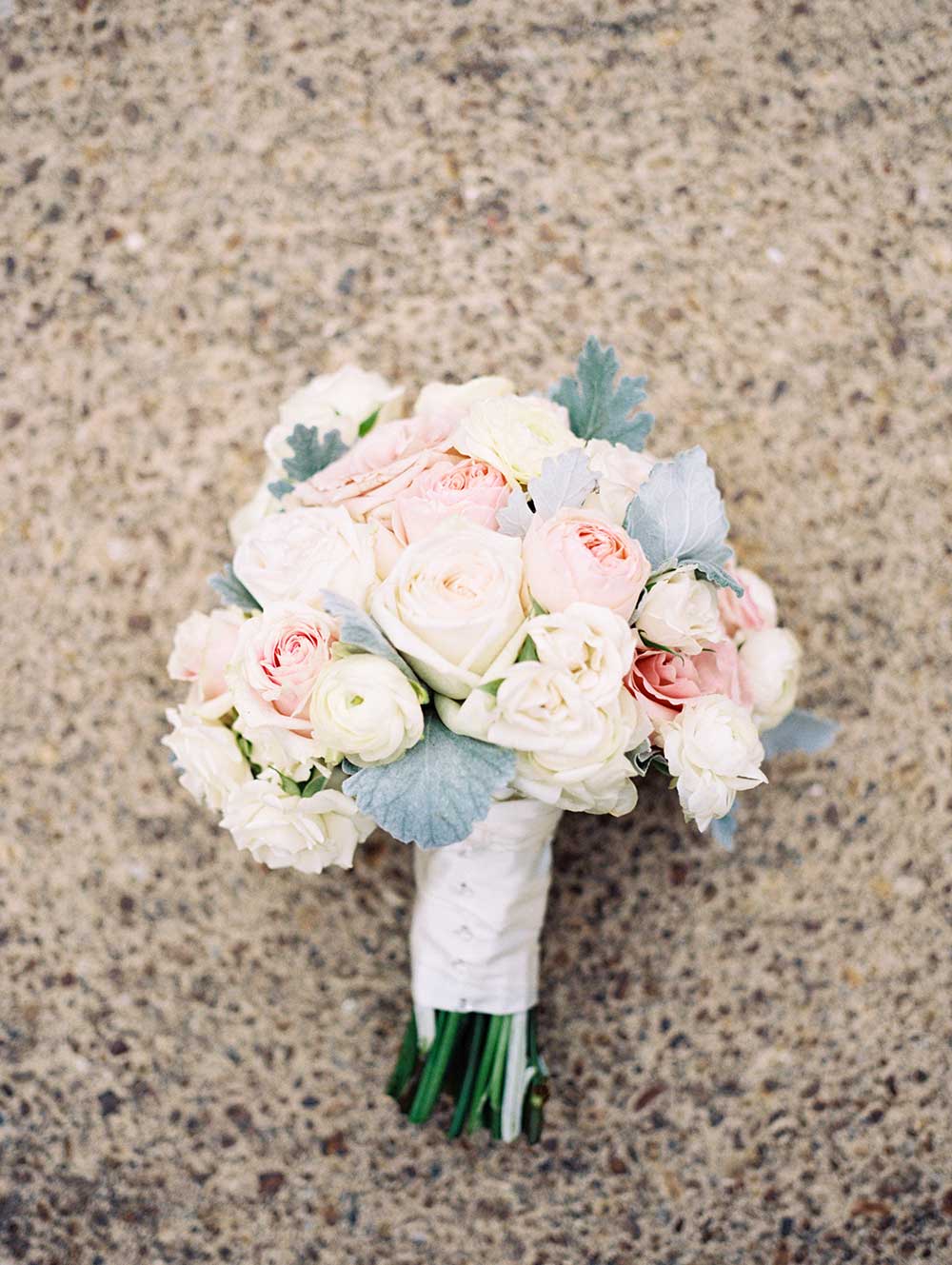The image depicts a bouquet of roses resting on a marble or granite countertop. The bouquet predominantly features white roses, interspersed with blush pink ones that are so light they are almost hard to distinguish from the white. The roses' stems are wrapped in a piece of white satin cloth and tied neatly, with the green stems extending from the bottom. Among the white and light pink petals, one tiny baby rose stands out. The leaves, painted with a whitish hue on one side, blend seamlessly with the flowers' soft colors. The overall composition and elegant wrap suggest it could be a bouquet used in a wedding, possibly by a bride, bridesmaid, or flower girl.